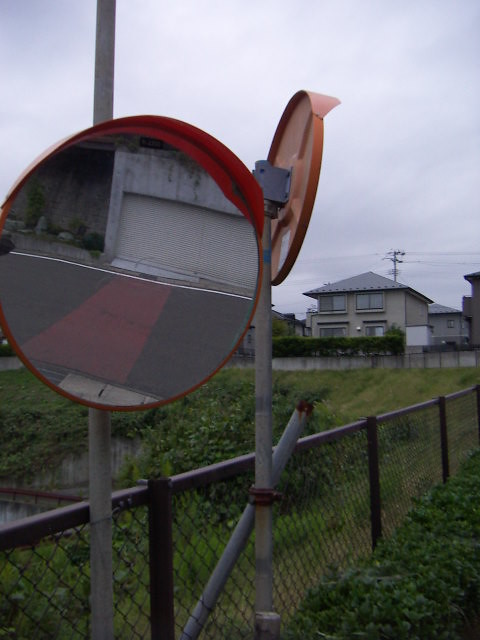In this overcast, daytime photograph, two large, round mirrors are mounted atop tall gray poles, rising approximately eight to ten feet above a black metal fence. Each mirror features a distinct red or orange shade above it. The mirror in the foreground reflects a paved, gray area marked with a striking red stripe and hints at the presence of a white garage door. Both mirrors are positioned to show different angles, likely serving safety purposes for the depicted road. Surrounding the mirrors is a field bordered by a chain-link fence, with various weeds and green plants to the right. To the left, there's a slight gully and some cemented areas with visible water. In the background, a beige two-story house with green bushes contrasts against the dreary gray sky, with telephone poles and wires strung overhead. The house faces the viewer and is set against a landscape of mixed greenery and additional residential structures.